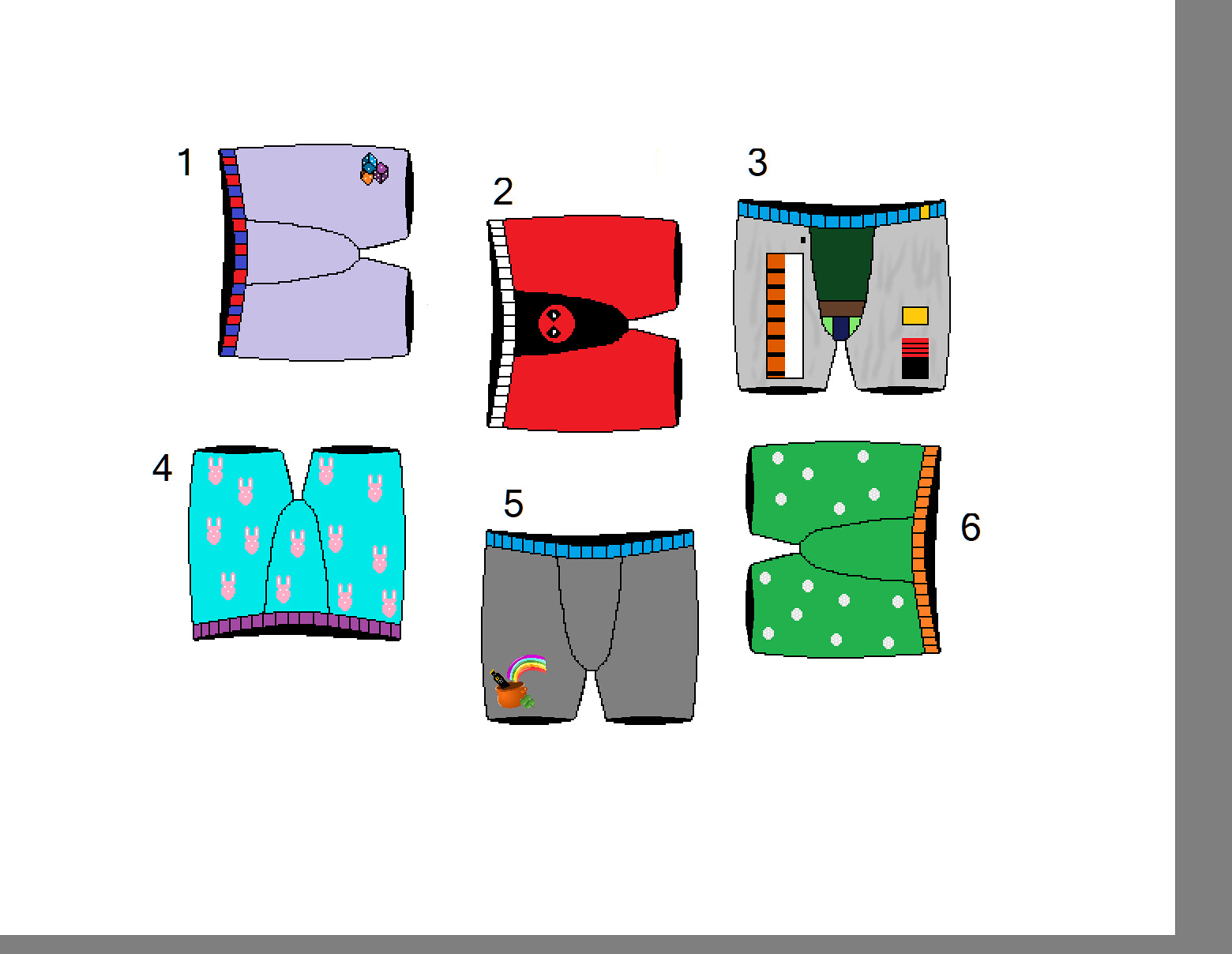The image depicts six cartoonish drawings of men's boxer briefs, each with unique designs and numbered one through six. The drawings are set against a white background bordered in gray on the right side and bottom. 

- **Number 1**: This pair features a light blue body with a red and blue waistband, adorned with three dice in various colors—blue, yellow, and purple.
- **Number 2**: Predominantly red with a black and white waistband, this pair has a black and red decoration at the crotch reminiscent of Spider-Man's face.
- **Number 3**: Displaying a gray body with a blue and yellow waistband, the crotch area is dark gray, blue, and light green, with several different colored rectangles.
- **Number 4**: This pair is light blue with a purple waistband, decorated with small rabbit faces sporting bunny ears.
- **Number 5**: Featuring a gray background and blue waistband, this pair includes a design at the lower left resembling a leprechaun's pot of gold with a rainbow and shamrock.
- **Number 6**: Green with white polka dots and an orange waistband.

All pairs are hand-drawn, possibly in a digital paint program, and laid out neatly with the numbers in black text above them.